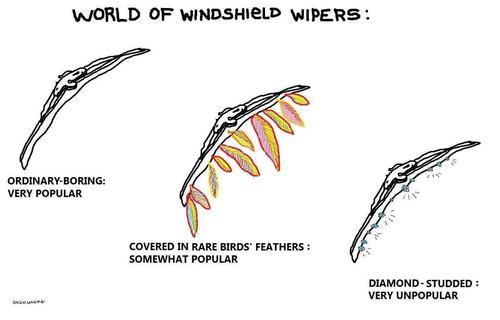This black and white graphic titled "World of Windshield Wipers" humorously categorizes three types of windshield wipers. At the top left, an ordinary and boring wiper is labeled as "Very Popular," depicted in a simple black line drawing. In the middle, a wiper "Covered in Rare Birds' Feathers" is labeled "Somewhat Popular," adorned with brightly colored feathers in shades of pink, yellow, teal, and red hanging below it. On the bottom right, a "Diamond-Studded" wiper, described as "Very Unpopular," is illustrated with small blue diamonds. The graphic combines detailed drawings with playful text to create a whimsical commentary on windshield wiper styles.